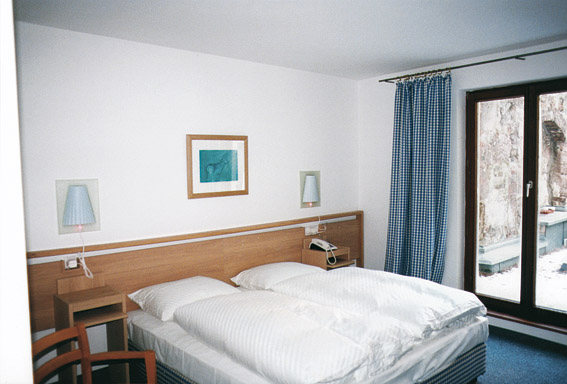This full-color indoor photograph captures a daytime scene inside a possible hotel room or bedroom. The room features white walls and a white ceiling. The centerpiece is a double-sized bed, possibly queen or king, adorned with white sheets, two pillows, and two blankets, all set against a long, rectangular wooden headboard. The headboard is flanked by two built-in wooden nightstands, each topped with a wall-mounted lamp and shade. Centered between the lamps above the headboard is a framed picture with predominantly blue tones. To the right of the bed, there are blue and white checked curtains, drawn open to reveal brown wooden French or sliding doors leading outside. The lower left corner of the image includes part of a brown chair, specifically its armrest. The blue carpet grounds the room, adding a touch of color, while the room overall exudes a crisp and tidy ambiance, ready to accommodate two guests.